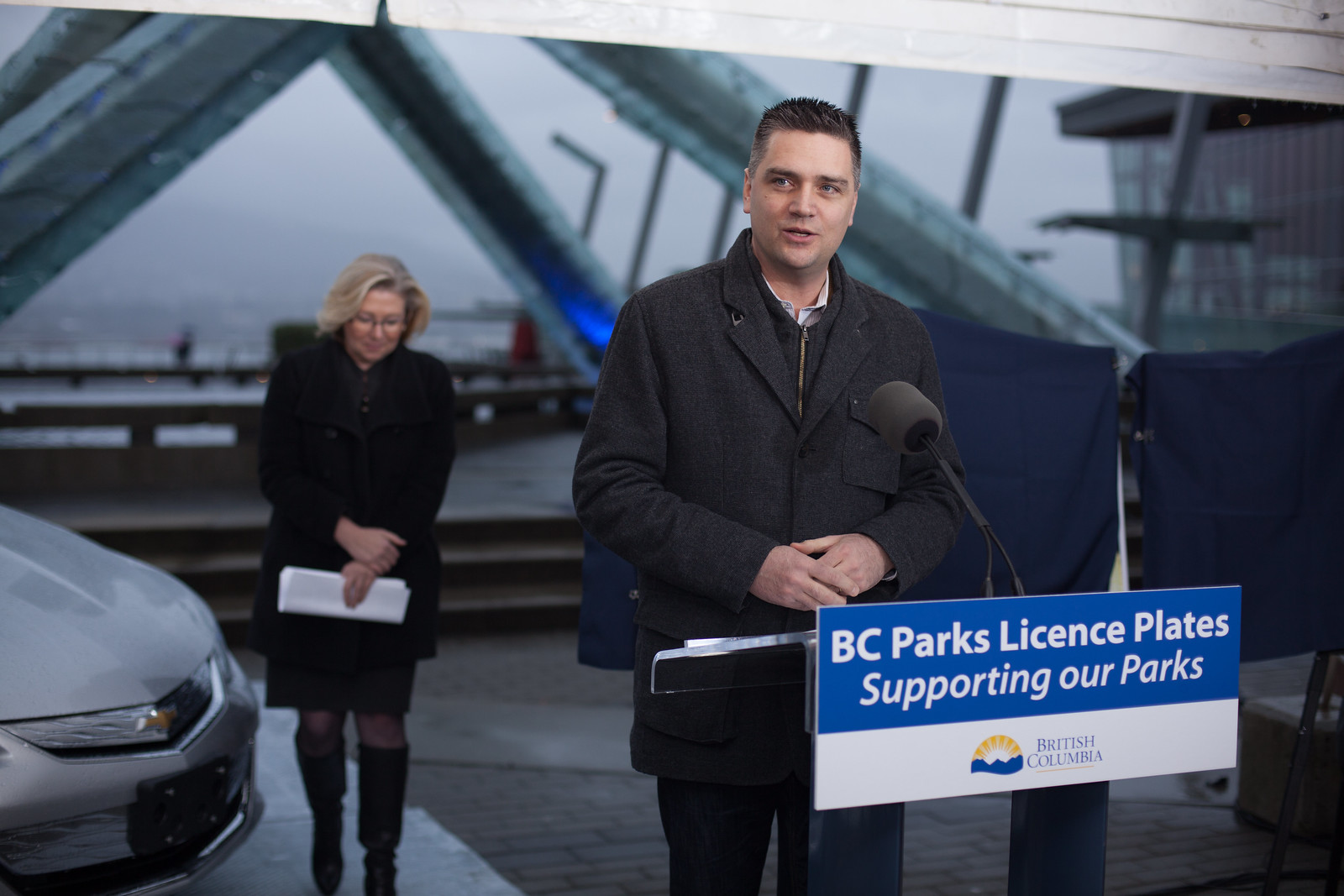In this image, a man is giving a presentation at a podium equipped with a microphone. The podium features a prominent blue and white sign that reads, "BC Parks License Plates Supporting Our Parks," with "British Columbia" written below. The man, who has short black hair, is dressed in a gray wool coat over a sweater, paired with jeans, and appears to be speaking or smiling. He stands outdoors on a concrete and brick pathway, under a gray, potentially rainy sky, which adds a cold atmosphere to the scene. To his left and slightly behind, a woman in a long black jacket and black boots is holding a white paper and looking down, seemingly cold. The front of a Chevrolet car is visible just to the side of her. The backdrop includes pillars of a building and a somewhat indistinct area that might be a pier or stage, contributing to the busy background.